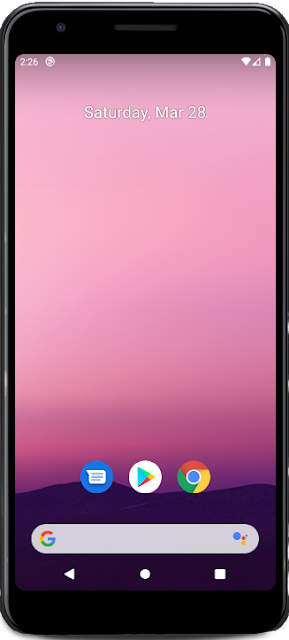A detailed caption for the provided image could be:

"A depiction of an Android smartphone with a distinctive design, possibly resembling an older iPhone model. The phone features a slim black frame with a visible camera at the top. The screen displays the device's interface, which indicates it is 2:26 on Saturday, March 28th, with the battery running low but a strong network connection. The background transitions from a pinkish hue at the top to black at the bottom, providing a striking contrast. Several apps are open on the screen, including a blue app icon, Google Play Store, and Chrome. At the bottom of the screen, the familiar Android navigation bar is present with a Google search bar, three dots, a triangle, a circle, and a square. The layout suggests this image might be used for web page advertisements or graphic design purposes, presenting a clear and detailed visual of an Android phone's interface."